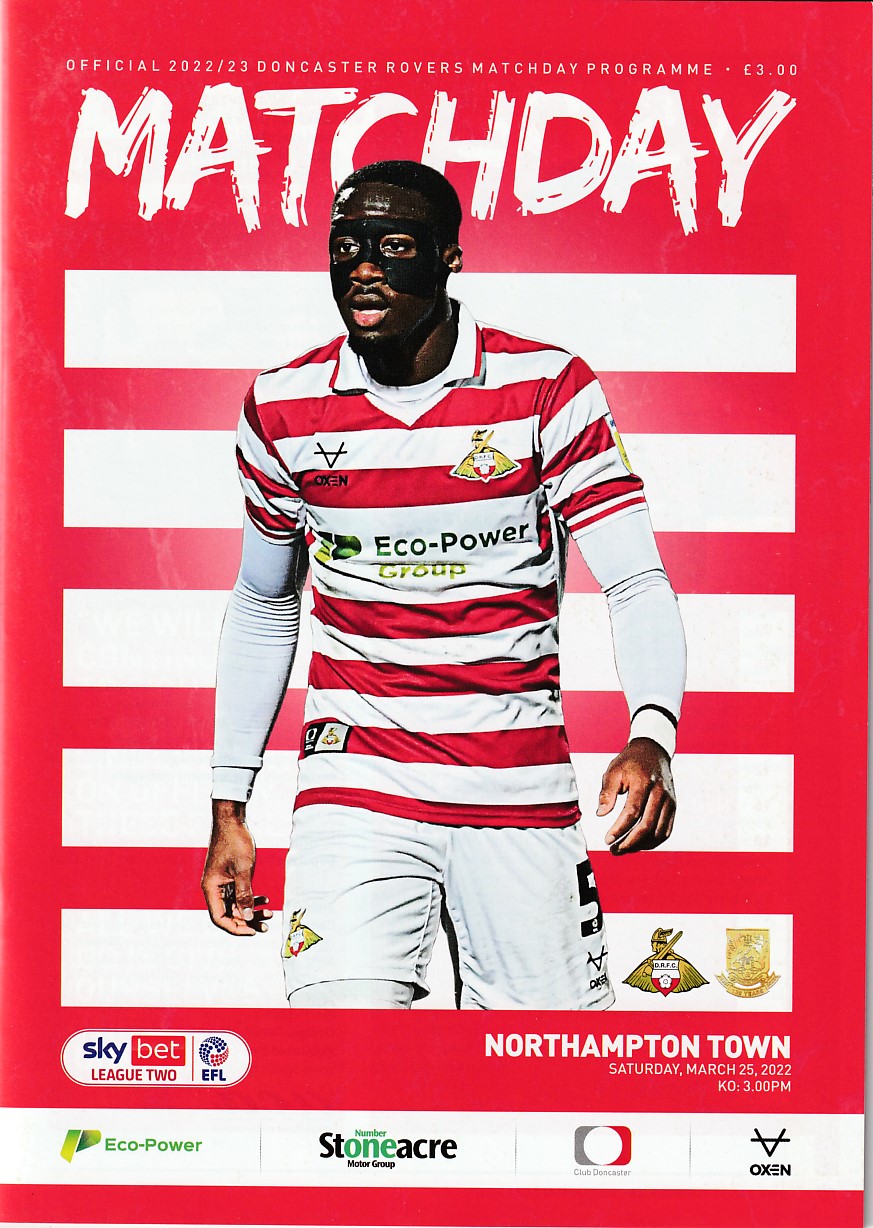The image depicts the cover page of the official 2022-23 Doncaster Rovers soccer program. This vibrant cover is designed with bold red and white horizontal stripes, set against a striking red background. At the top of the page, "MATCH DAY" is prominently displayed in large, white lettering, with "Official 2022-23 Doncaster Rovers Program" written above it in smaller text, along with the price, indicated as "£2".

Dominating the central area of the cover is an image of a black soccer player wearing the distinctive red and white striped jersey of Doncaster Rovers, featuring the sponsor insignia "Eco-Power" on the front. His arms are extended down his sides, and he is also wearing white shorts. Below his left hand, the Doncaster Rovers team logo is prominently displayed.

Beneath the team logo, the details of an upcoming match are provided: "Northampton Town, Saturday, March 23rd, 2022, Kick-off 3 p.m.". To the left of these match details, various sponsor logos are visible. The familiar "Sky" logo is positioned within a white oval containing the word "BET". At the bottom of the page, additional sponsors are listed against a white background, including "Eco-Power" and "Stoneacre". There is also a square with a red right side and a gray left side, although the name within it is obscured. Adjacent to that is an inverted "A" accompanied by the letters "O R E N", indicating another program and team sponsor.